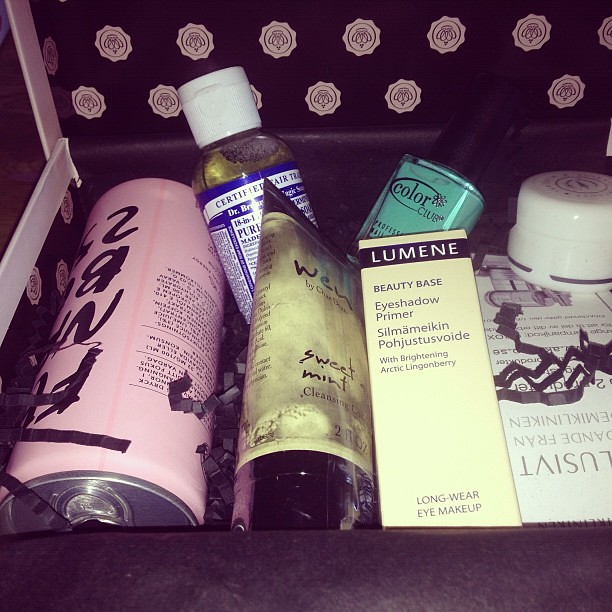The image depicts a decorative display box containing a variety of cosmetics, presented as a comprehensive care package or gift set. The box has dark interior walls, either black or very dark navy, adorned with pink pastel circular logos featuring a black crown outline on the back and sides. The edges are trimmed with pink or pinkish taupe taping. Within, the box holds six distinct beauty items and is filled with black shredded paper for padding.

From left to right, the contents include:
1. A pink cylindrical can, reminiscent of an energy drink can, bearing black text that remains unreadable.
2. A clear bottle with a white cap, labeled with some form of certification.
3. A tube with a black cap labeled "WEN Sweet Mint Cleansing Cream."
4. A long, rectangular white box labeled "Lumene Beauty Base Eyeshadow Primer," with additional details in a foreign language about its long-wear properties.
5. A glass nail polish bottle with a mint green tint and black cap, labeled "Color Club" along with a floral logo.
6. A small white jar.

The box also contains a brochure, contributing to the perception that it’s a thoughtfully arranged, lovely gift set, ideal for a variety of cosmetic needs.